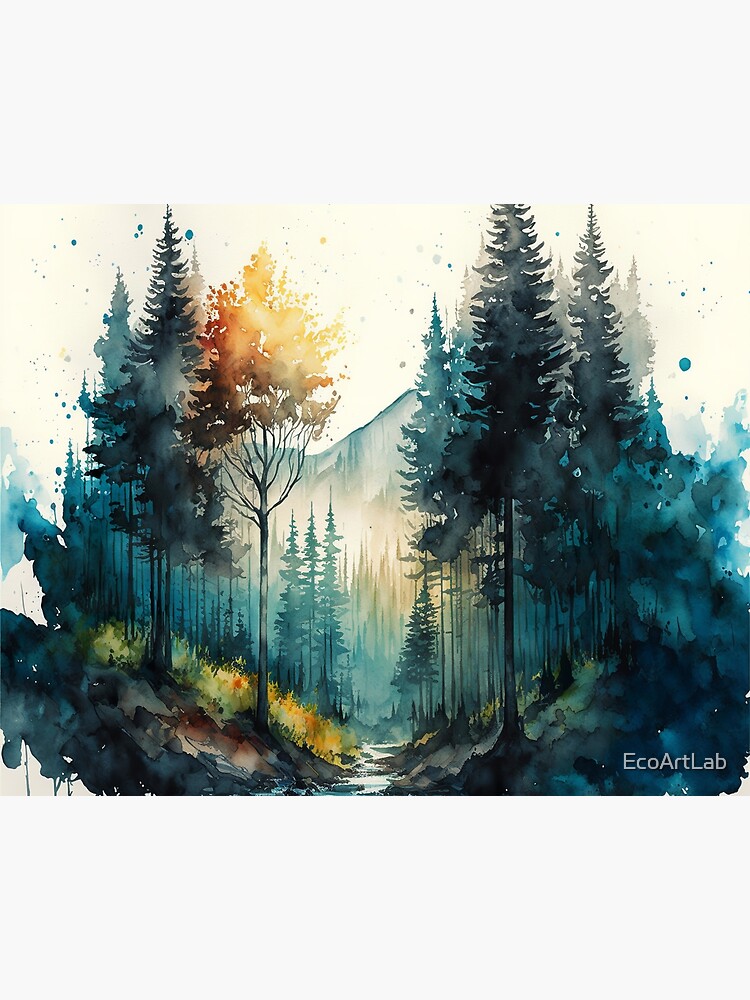This close-up photo captures a small square watercolor painting depicting a serene forest valley. The forest is populated with tall trees in varying shades of blue, green, and deep orange, with occasional black tones lending a sense of depth. A golden, sunlit tree on the left adds a touch of warmth. A shallow creek flows gently through the center-bottom of the scene, meandering through grassy hills that ascend into a valley. These hills are painted in harmonious shades of green, yellow, and brown. Conifer trees stand tall along the slopes, some cloaked in a faint mist near their bases, while a towering mountain forms a majestic backdrop, lightly shrouded in fog. The sky above is a blend of white and yellow hues, transitioning into an abstract splattering of teal dots at the top, giving a melting, ethereal effect. The painting rests on a lighter white background, and a subtle white watermark in the bottom right corner reads "Echo Art Lab."